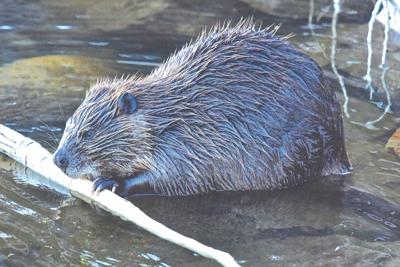A detailed digital painting depicts a beaver in shallow, muddy water, approximately four to five inches deep. The beaver, facing left in an almost full profile, is chewing on a light tan stick. Its wet fur is a mix of brownish-gray, dark chocolate brown, and a few streaks of black, giving it a spiky appearance. The animal has distinctive features, including black front paws with white claws, round black ears, and a dark gray nose. Its black eye is surrounded by a thin circle, and the white fur contrasts subtly with the overall darker hues of the beaver.

The scene is rich with detail: it has a granitic background with stones visible both within and above the water. Vines hang down into the water on the right-hand side of the image, while thin ribbons of white float in the upper right corner. The bright sunlight illuminates the stick in the beaver's mouth, casting a white glow. The setting, possibly outdoors or in a zoo environment, captures the beaver's natural habitat in a close-up landscape orientation, accentuating the muddy, rocky puddle and the wet lower body of the beaver.